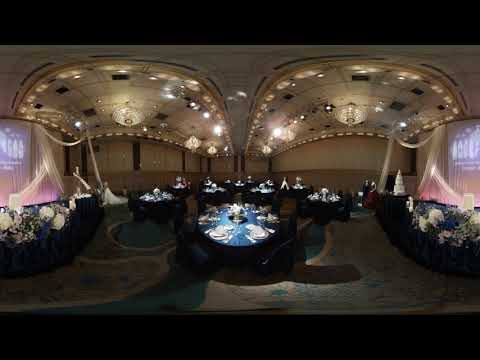The image depicts a dimly lit, expansive banquet hall, elegantly set for a high-end event such as a wedding or anniversary. The room features a prominent central table adorned with a blue tablecloth and ornate place settings, clearly designed for fine dining. Surrounding this main table, there are smaller tables similarly set up, all decorated with lavish floral arrangements, including large white flowers flanking the central table and smaller bouquets as centerpieces on each dining table. 

Overhead, the ceiling boasts ornate light fixtures, including two visible chandeliers among other smaller lights that cast a warm, golden glow. The architecture of the ceiling also hints at potential mirrors or reflective surfaces, adding to the room’s grandeur. The sides of the main table are framed by what appear to be divider walls or sheer curtains with reddish and purplish hues, possibly indicating screens or stages. 

In the background, particularly on the right-hand side of the room, there is a wedding cake, with two individuals nearby, one of whom is clad in a striking red dress. The venue gives off an opulent, mirrored aesthetic, enhancing its luxurious and spacious feel, perfect for a significant celebration.